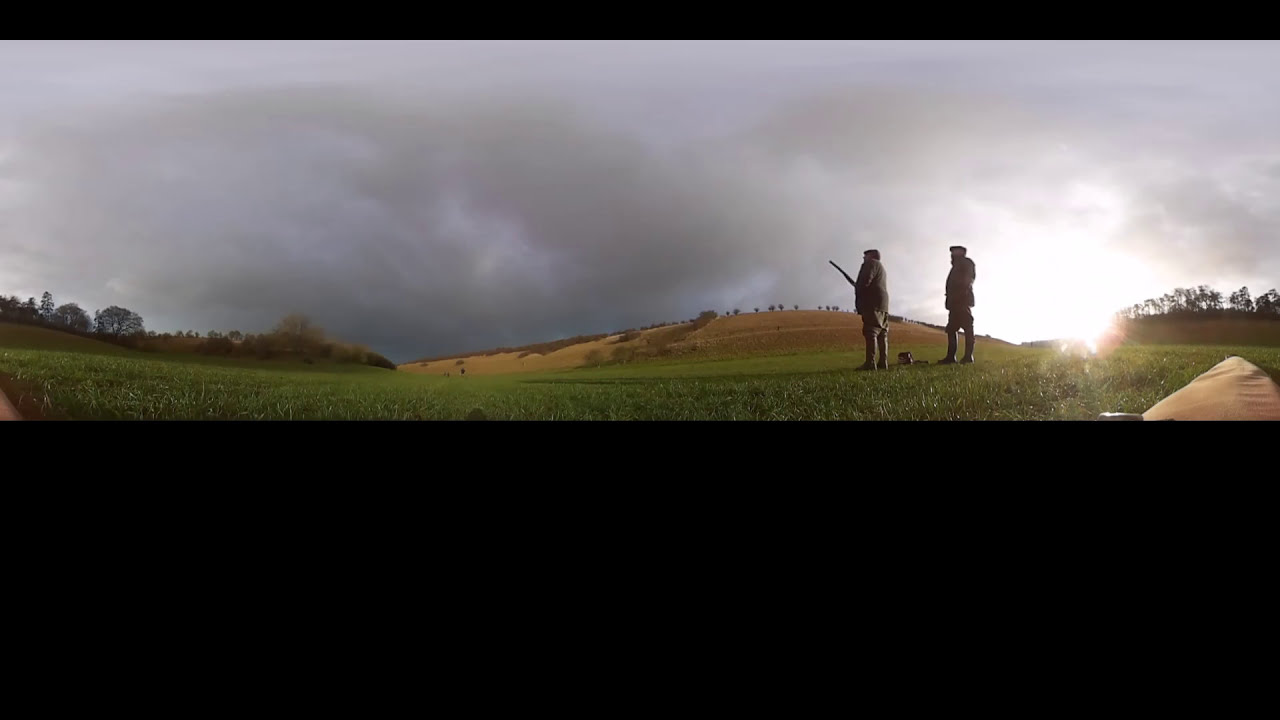The image captures an outdoor panorama featuring two silhouetted men, possibly hunters, standing in a green field under an overcast sky with gray clouds. The lower 40% of the frame is dominated by a solid black horizontal line, while the sun low in the sky peeks through the clouds on the right-hand side, suggesting it's late evening. Both men are positioned towards the right-third of the picture, gazing to the left. One man seems to be holding a rifle, indicating they might be hunting. There's a dog positioned behind them, either sitting or lying down. The background showcases a gently sloping hill with tan grass, dotted with clusters of trees on both ends. The overall scene exudes a quiet, contemplative moment in a peaceful outdoor setting.